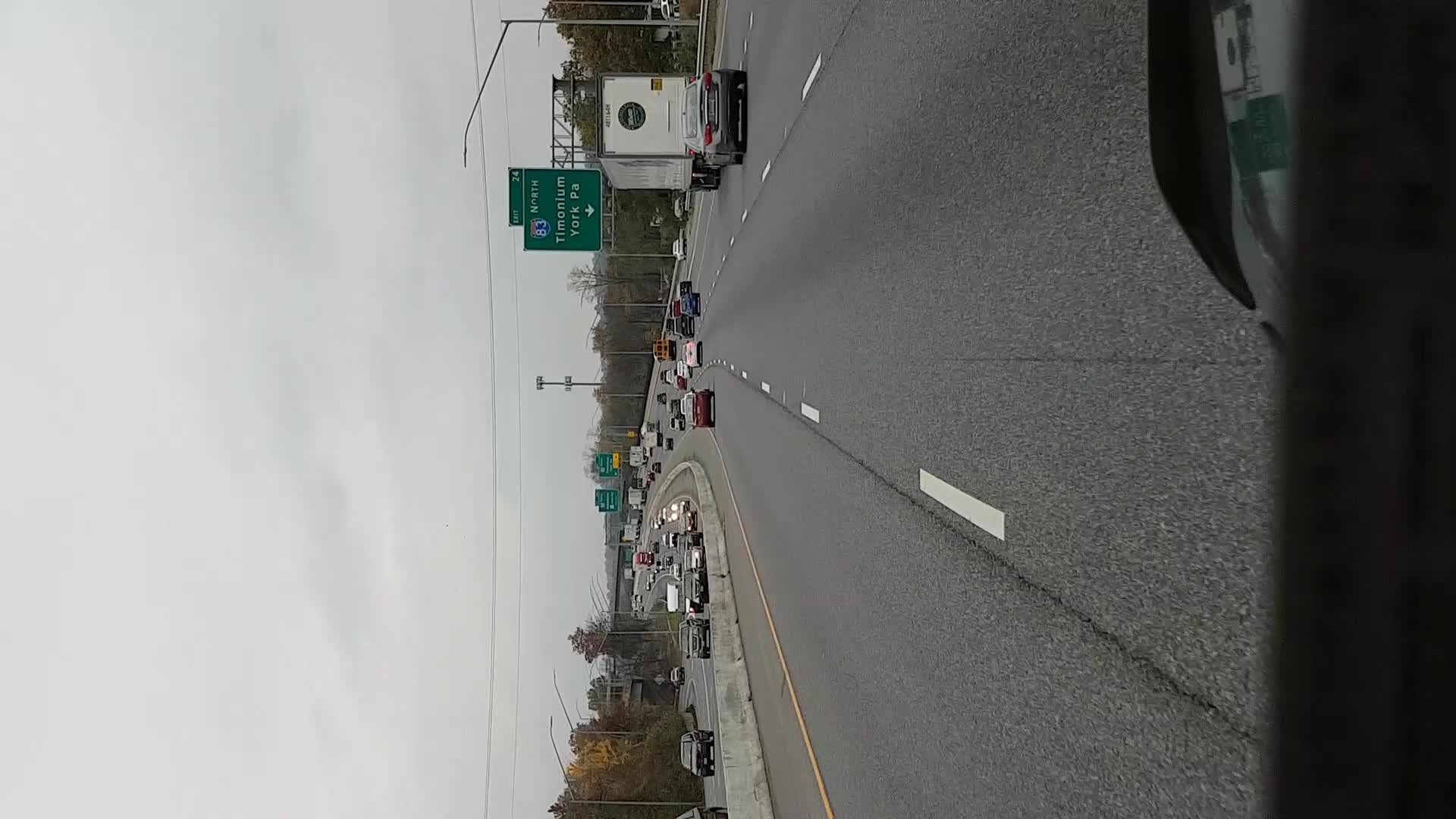A sideways cityscape image taken through a car windshield, showcasing a bustling, gray highway under an overcast sky. The rotated picture captures heavy traffic on a four-lane road, with a concrete barrier separating lanes moving in the opposite direction. In front of the car, there is a small sedan followed by a white semi-truck. Prominently featured is a green highway sign, indicating "83 North" and "York, PA," along with an exit number 24 and directional arrows. Further up the road, additional green highway signs are visible, guiding drivers through the busy lanes. The sides of the highway are lined with trees, bushes, and glimpses of a cityscape. This detailed scene, viewed from a low vantage point within the vehicle, emphasizes the chaotic yet structured nature of urban highways.